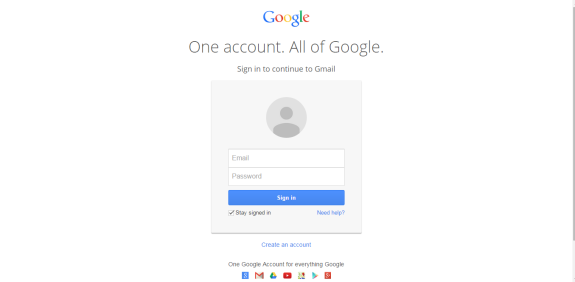The image is a screenshot of the Google sign-in page. The background is predominantly white. At the top, the Google logo is displayed with the letters in distinct colors: the "G" in blue, "o" in red, the second "o" in yellow, "g" in blue, "l" in green, and the final "e" in red. Below the logo, the text "One account." is written in black with the 'O' in uppercase.

Further down, another line of black text instructs, "Sign in to continue to Gmail," with 'G' capitalized. Following this, there's a light gray rectangle with evenly tapered sides. Inside this rectangle, there's a slightly darker gray circle featuring two additional darker circles within it, partially depicting a creative person though the bottom part is cut off.

Below this section, there are three rectangular fields: the first two are outlined in gray and have a white fill. The first rectangle has the placeholder text "Email" in light gray, indicating where users should enter their email addresses. The second rectangle has the placeholder text "Password" in light gray, marking it as the password entry field. The third rectangle is a blue button with white text that reads "Sign in."

Beneath the sign-in button, there is a checkbox labeled "Stay signed in" with a checkmark in black next to it. Below the checkbox, there is a link in blue text that reads "Need help?" and another link that says, "Create an account." At the very bottom, in black text, the phrase "One account. All of Google." is written.